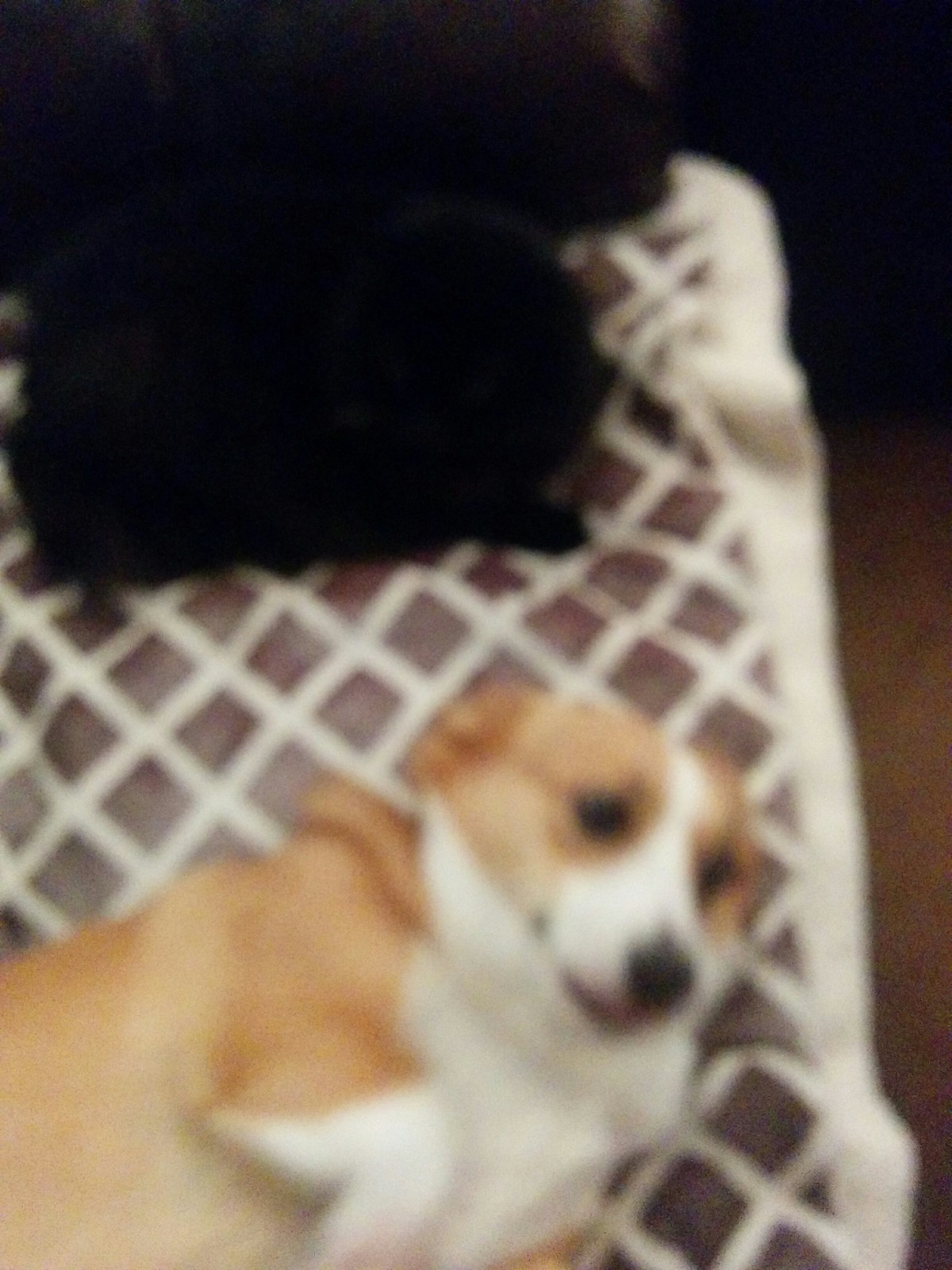This blurry photo, presumably taken inside someone's living room or bedroom, depicts a cozy scene from an elevated viewpoint. Although the image quality is fuzzy, you can discern a piece of furniture, likely a bed or a couch, covered with a blanket featuring a repeating pattern of small brown diamonds on an ivory background. Nestled on this blanket are two dogs. The dog at the top of the frame is shrouded in shadows, making it difficult to identify its breed beyond its black fur. At the bottom of the frame lies a light brown and white corgi, comfortably resting with its feet up and facing to the right. The corgi's distinct white markings can be seen on its nose, extending between its eyes.